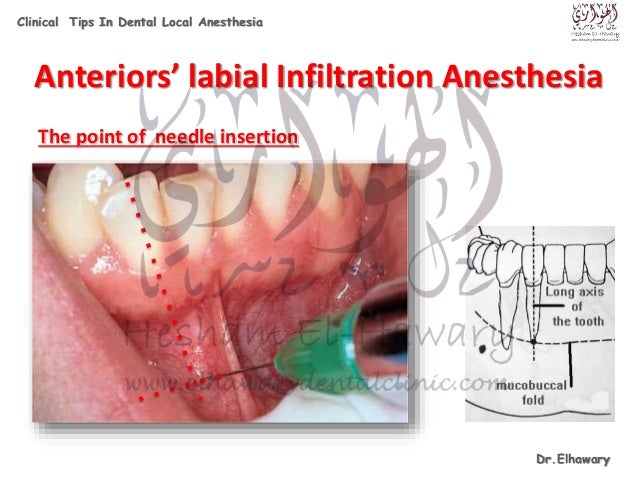The image appears to be a slide from a PowerPoint presentation related to dental procedures. The background is entirely white. In the top left corner, black text reads "Clinical Tips in Dental Local Anesthesia," and in the top right corner, there is a logo in Urdu or Persian. Below, in large red letters, the heading states "Anteriors Labial Infiltration Anesthesia." Under this, a red underlined subheading reads "The Point of Needle Insertion." The central portion of the slide features a detailed color image of a needle being inserted into the gum line just below the teeth, illustrating the procedure. To the right of this, there is a smaller black-and-white diagram showing a close-up of teeth, highlighting the long axis of the tooth and the mucogingival fold. At the bottom right of the slide, the name "Dr. Hesham Alhawry" is displayed, along with his website, "www.heshamdentalclinic.com." The same Urdu or Persian logo appears as a watermark on the image.